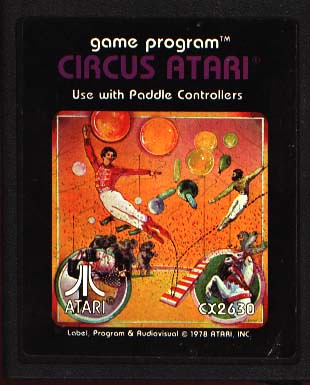This image is a detailed photograph of a game box for an old-school Atari console game titled "Circus Atari." The prominent black outline frames white lettering at the top that reads "Game Program TM," followed by "Circus Atari" in a bold, larger purple font. Below this, in white letters, it instructs to "Use with Paddle Controllers," indicating the game's compatibility with the specialized controllers rather than the typical joysticks.

The center of the box features an orange square with a white outline, depicting a lively circus scene. Within this square, a performer in a red top, white pants, and red boots is illustrated flying off to the left, seemingly launched from a teeter-totter-style springboard. This red and white-striped board is anchored on an orange ground. Another acrobat dressed in a green top and white pants is depicted gliding downwards in the scene. Floating throughout the image are round, orange and lighter orange balls, resembling balloons or spheres adding to the circus ambiance.

More circus elements are scattered within the illustration: a white horse with a red headdress and bridle, three elephants standing on their hind legs, and other small, unclear elements that evoke the bustling, colorful setting of a circus. 

In the bottom corners of the orange square are two circles. The lower left circle contains the classic Atari logo, while the lower right displays the text "CX2630." Below the entire image in small text, the words "Label Program and Audiovisual 1978 Atari Inc." mark the game's copyright and production details. This vividly detailed game box sits against a black background, making all elements distinctly stand out.